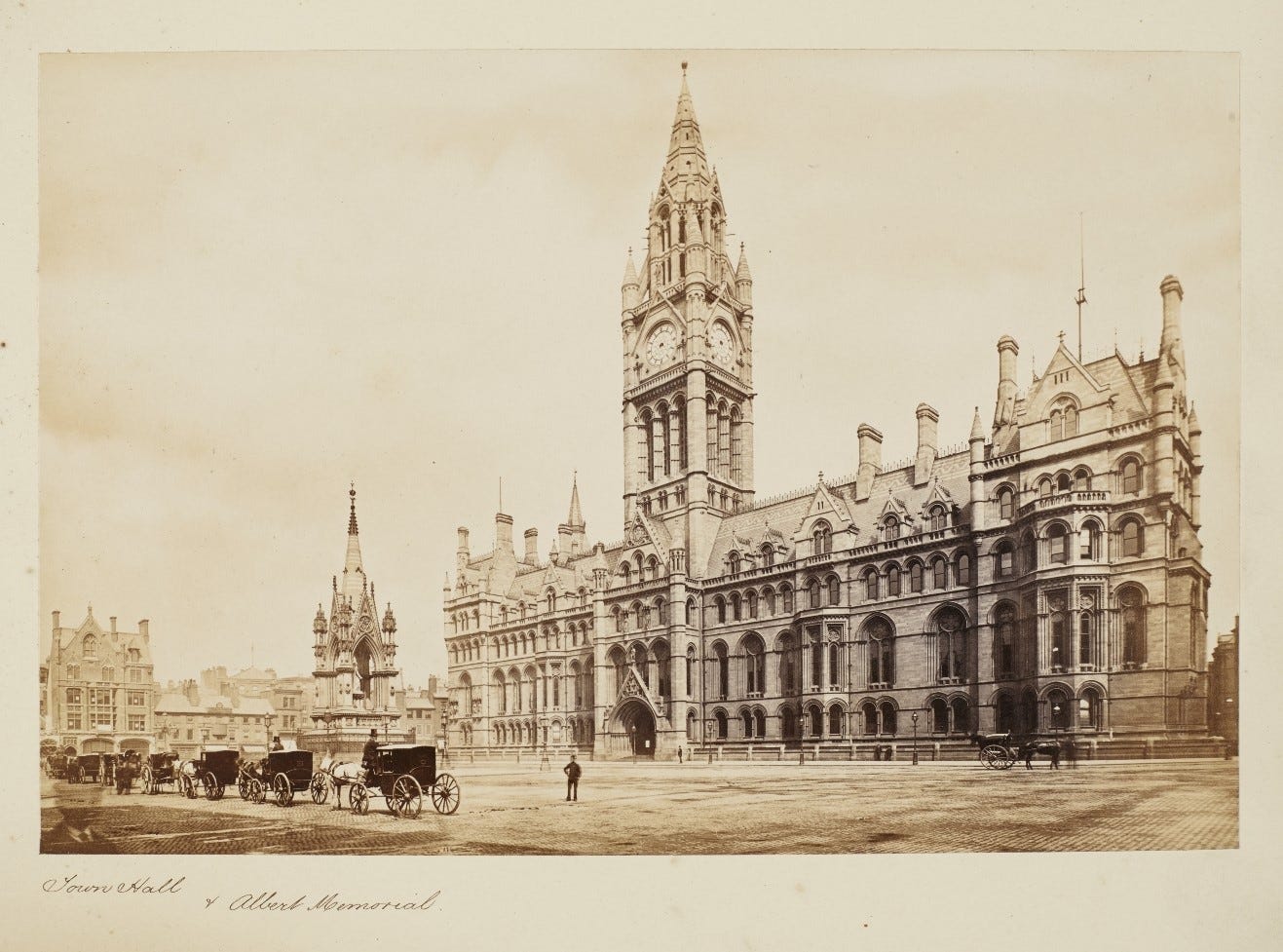The sepia-toned, black-and-white image, possibly a vintage drawing or photograph, showcases a bustling late 19th-century European street scene. Dominating the background is a grand, multi-storied town hall featuring a striking clock tower topped with a tall spire. Architectural details such as arched doorways and windows, along with decorative columns, are prominent. To the left of the clock tower, the Albert Memorial can be identified among the cluster of buildings. The wide street in the foreground is alive with activity, including several horse-drawn carriages lined up, their drivers wearing stovepipe hats. A man stands in the middle of the street, adding to the historical ambiance of the image. Notably, the aged appearance of the photo, with its yellowed and sepia tones, suggests it could be a historically significant illustration or a postcard. At the bottom left corner, the text reads "Town Hall, Albert Memorial," providing context to the location and landmark depicted.